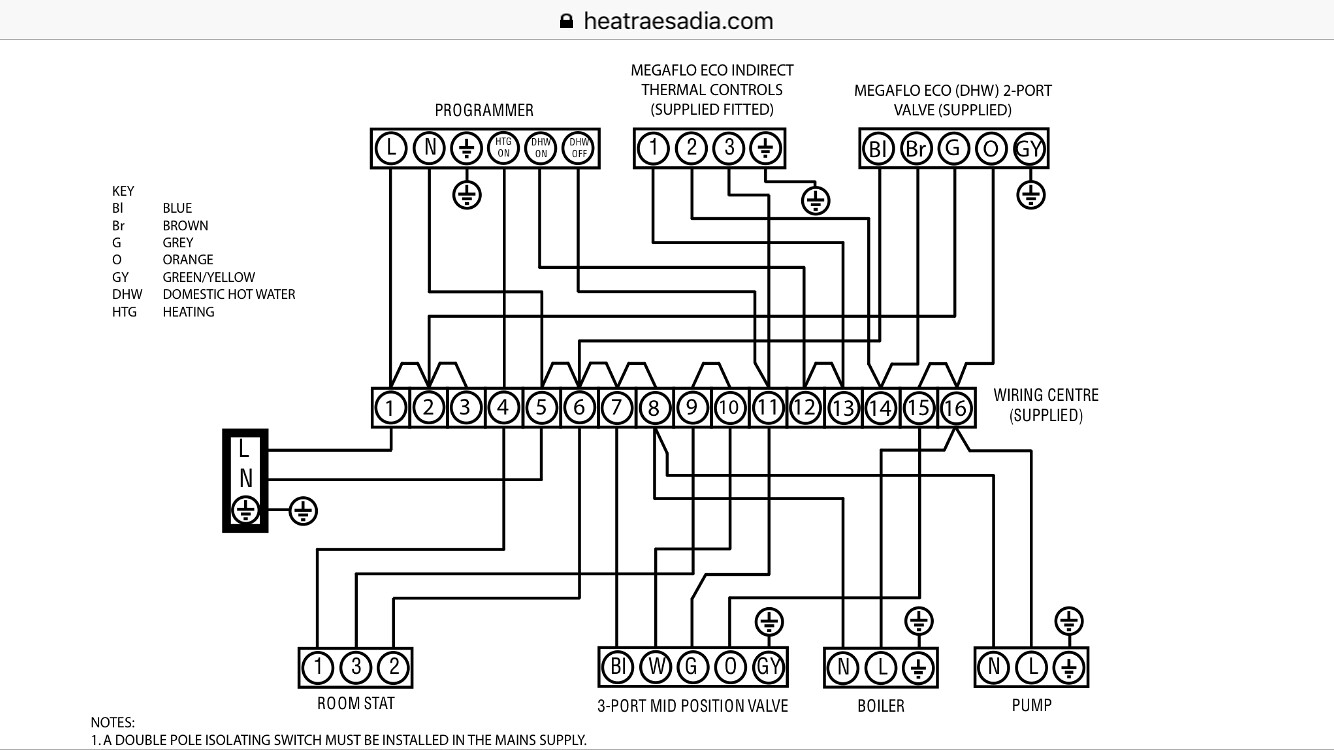This black and white wiring diagram, possibly for a water heater or another type of residential heater, features a comprehensive and intricate layout of components. The diagram includes numerous letters and numbers enclosed within circles, which are interconnected by lines running throughout the schematic. 

At the top of the diagram, a URL is prominently displayed: [heatresadia.com](http://heatresadia.com). To the left, a key explains the abbreviations used in the diagram: BL (Blue), BR (Brown), G (Gray), O (Orange), GY (Green Yellow), DHW (Domestic Hot Water), and HTG (Heating). These abbreviations appear in various circles throughout the diagram.

The bottom of the diagram includes a notation: "A double pole isolating switch must be installed in the main supply."

At the top of the page, there are three rectangles, each with a circle at its center. One notable feature is a lengthy rectangle divided into squares, each containing numbers 1 through 16, labeled "wiring center supplied."

The bottom section of the schematic features four more rectangles, each containing circles that are labeled with different numerical and alphabetical designations. These rectangles are labeled as follows:
1. Room Stat
2. Three Port
3. Mid Position Valve
4. Boiler and Pump

Overall, the diagram is a detailed and organized guide to the wiring of a heating system, with clearly labeled components and helpful keys to aid in understanding the layout and connections.